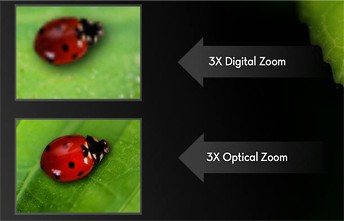The image showcases a comparison between two camera zoom types, featuring two rectangular inserts positioned on the left side. Each insert contains a photograph of a ladybug with a red body, black spots, and a black head, resting on a green leaf. The photographs highlight the differences between 3x digital zoom and 3x optical zoom, as indicated by white text on light gray arrows pointing from the right side towards each ladybug. The top insert, labeled "3x digital zoom," displays a blurred image, making the details of the leaves and the ladybug indistinguishable. In contrast, the bottom insert, labeled "3x optical zoom," shows a vivid, crisp, and sharper image. The overall setting of the image is technologically oriented, with a focus on camera capabilities and macro photography. The background is black, with a hint of green in the top right corner, contributing to the emphasis on the subject matter.